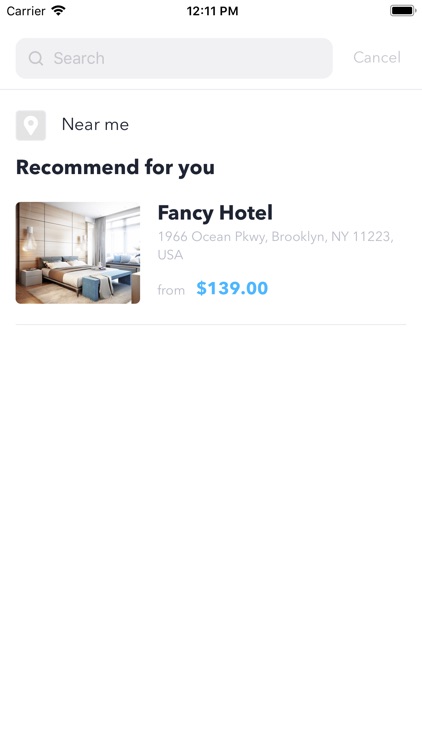This image is a screenshot of a mobile phone displaying hotel information against a pure white background. At the very top of the screen's header, the text "Carrier" is displayed in black on the left side, accompanied by a fully filled black Wi-Fi icon. Centrally positioned, the time reads "12:11 PM" in black text. On the far right, a fully charged battery icon is depicted in black.

Directly under the header is a light gray search bar featuring a darker gray magnifying glass icon followed by the word "Search." To the right, outside the search bar, there is light gray text that says "Cancel." A thin gray line separates this section from the main content of the page below it.

The primary information block starts in the top left with a gray square that has rounded corners. Inside the square is a white geographic pin, and next to it, "Near Me" is written in black text. Below this, in bold black letters, the text reads "Recommended for You." The hotel name "Fancy Hotel" follows. To the left of this text block, there is an image of a hotel room featuring a bed, a blue table at the foot of the bed, a wooden wall, and a brightly lit white window on the right.

Underneath "Fancy Hotel," the address is listed in light gray text: "1966 Ocean Parkway, Brooklyn, New York 11223 USA." Below the address, it states "From" followed by the price in blue, "$139.00." This section is concluded with another thin gray line, separating it from the remaining empty negative space at the bottom of the screenshot.